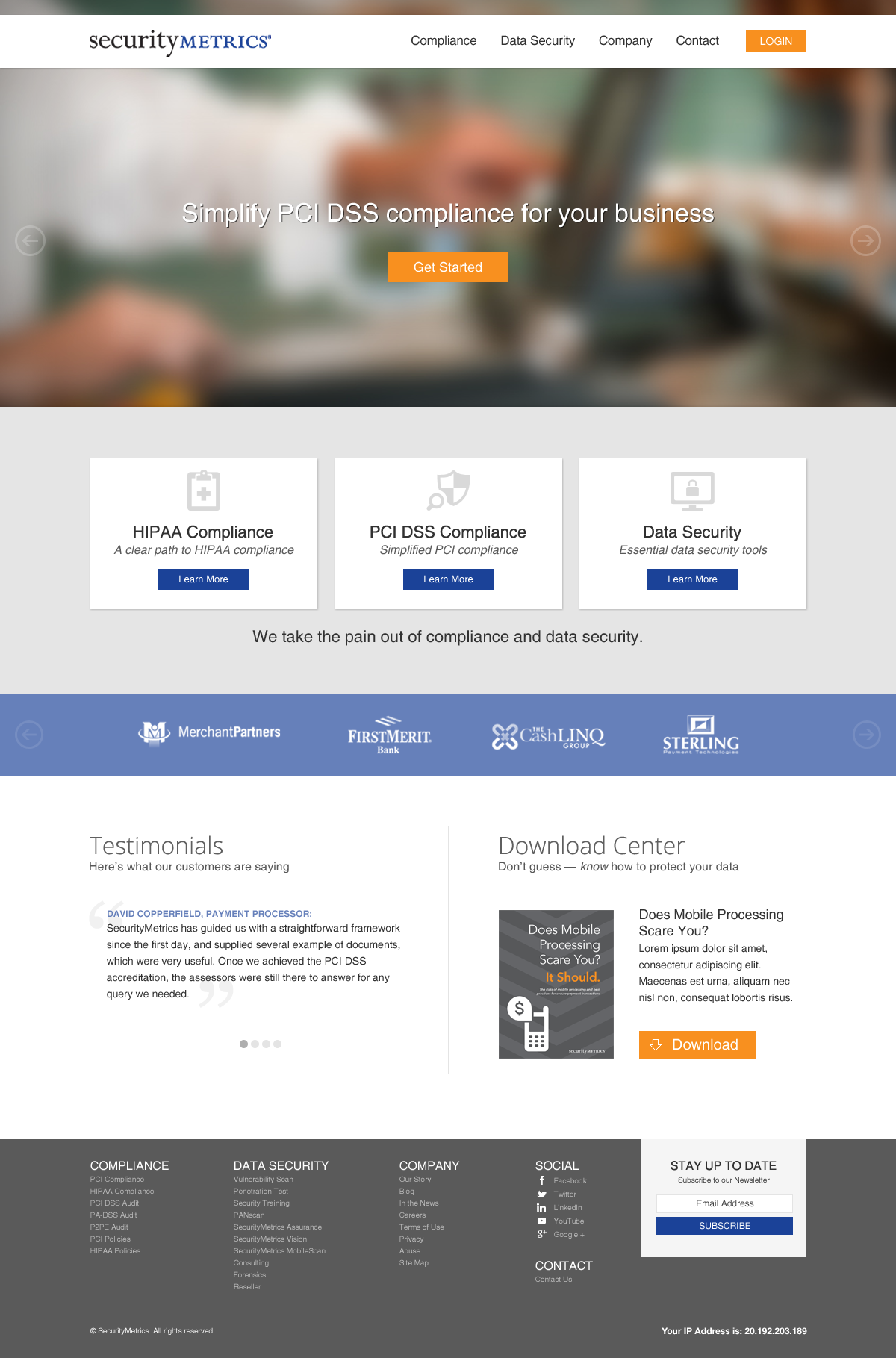The image depicts a website for "Security Metrics," featuring the word "Security" in dark blue and "Metrics" in a lighter blue. Positioned to the right are menu options written in black: "Compliance," "Data Security," "Company," and "Contact." Adjacent to these words, there's an orange rectangle with white text reading "Log In." 

Directly below this header section, there is a blurry image that somewhat reveals a hand pointing at a laptop. Superimposed on this image are white words stating, "Simplify PCI DSS compliance for your business." Below this message, there's another orange rectangle labeled "Get Started."

Further down, the webpage showcases three distinct boxes with the following details:
1. The leftmost box contains a gray clipboard icon accompanied by black text stating "HIPAA compliance." Within this box, there's a blue rectangle button.
2. The rightmost box features an image of a laptop with a lock on its screen, with "Data Security" written in black text. This box also includes a blue rectangle button.
3. Positioned somewhere on the page is an illustration of a cell phone with a chat bubble emerging from it, containing a dollar sign.